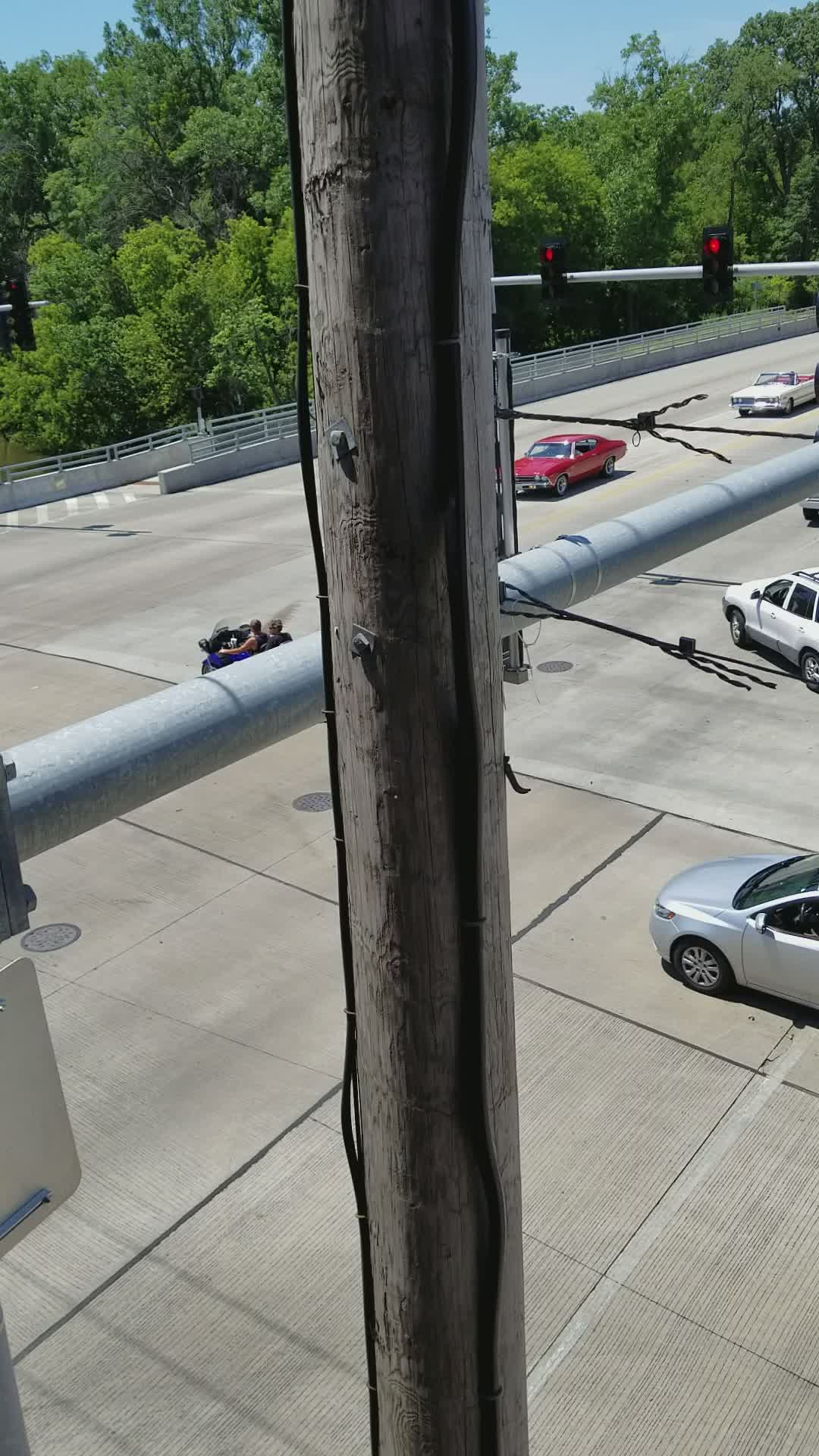The image prominently features an old-fashioned telephone pole, composed of weathered brown wood studded with metal fixtures, positioned vertically in the foreground above a parking lot. Multiple wires extend out from the pole, particularly branching off to the right. In the background, a bustling urban street with six visible lanes unfolds. A red traffic light governs the scene, where several slightly old-fashioned cars from the 1980s, including a red car and a white car, navigate the thoroughfare. The telephone pole stands as the focal point amidst the vibrant cityscape, providing a glimpse into the urban environment beyond.